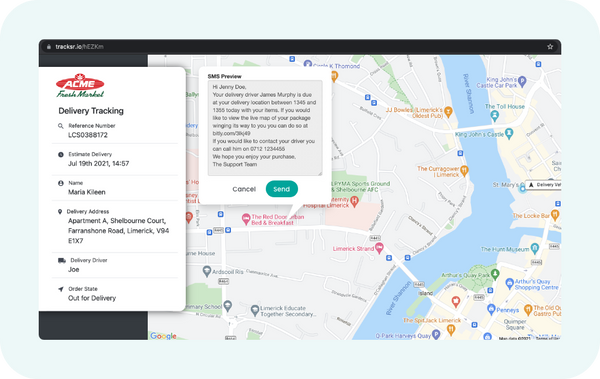**Caption:**  
The image depicts a Google Maps interface used for delivery tracking by ACME Fresh Market, a grocery store. The map shows a detailed view of a downtown area bisected by a river, with various streets and landmarks clearly marked. Numerous orange pins dot the map, identifying pubs and restaurants, while other colored pins indicate significant locations such as Toll House, King John's Castle, and Blue Castle. The King John's Castle car park is denoted with a "P" for parking.

On the right side of the screen, there is an SMS preview message addressed to Jenny Doe, informing her that the delivery driver is scheduled to arrive at a specified time, with options to cancel or send the message in a teal button with white writing.

To the left, a dialog box is present displaying a red oval ACME logo crowned with lights, followed by "Fresh Market" in green and "Delivery Tracking" in black. It includes a reference number for order issues, an estimated delivery time of July 19, 2021, at 14:57 hours, the customer's name, Maria Killeen, her delivery address at Apartment A, Shelbourne Court, and the delivery driver named Joe. The order status is listed as "Out for Delivery," emulating services like DoorDash.